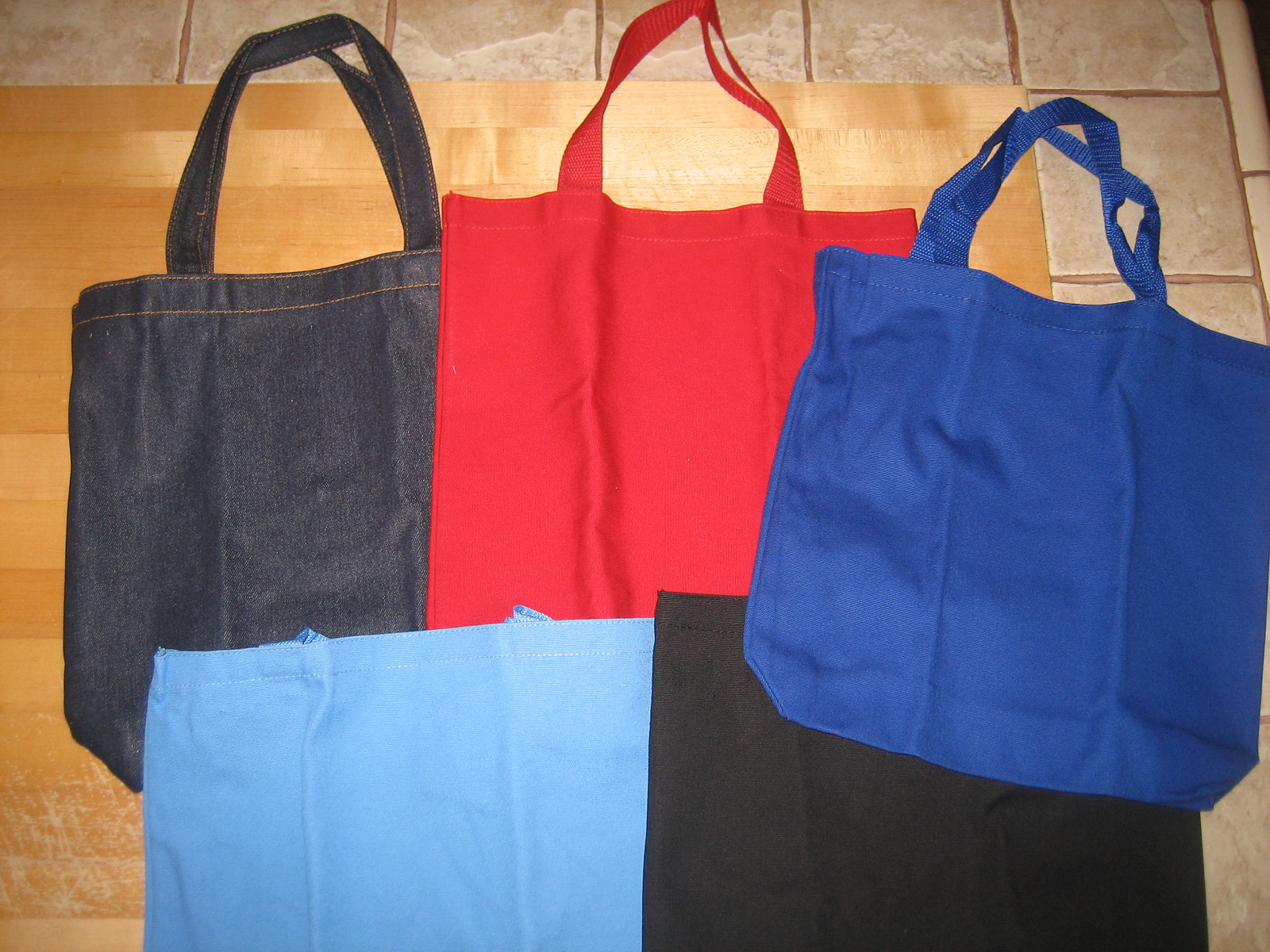This photograph, taken from a top-down angle, features five empty cloth tote bags arranged on a wooden tabletop, which sits on a white ceramic tile floor. The bags are spread out, slightly overlapping each other. At the top left, there's a bag crafted from denim with distinct dark grayish-blue and yellow stitching. In the middle is a plain red bag with two visible straps at the top. To its right, there is a royal blue bag with thin extended straps. At the bottom, there are two more tote bags: a light blue one on the left and a plain black one on the right. The two bags at the bottom have their handles tucked in and are less prominent in the frame. All the bags appear solid-colored with no additional designs.